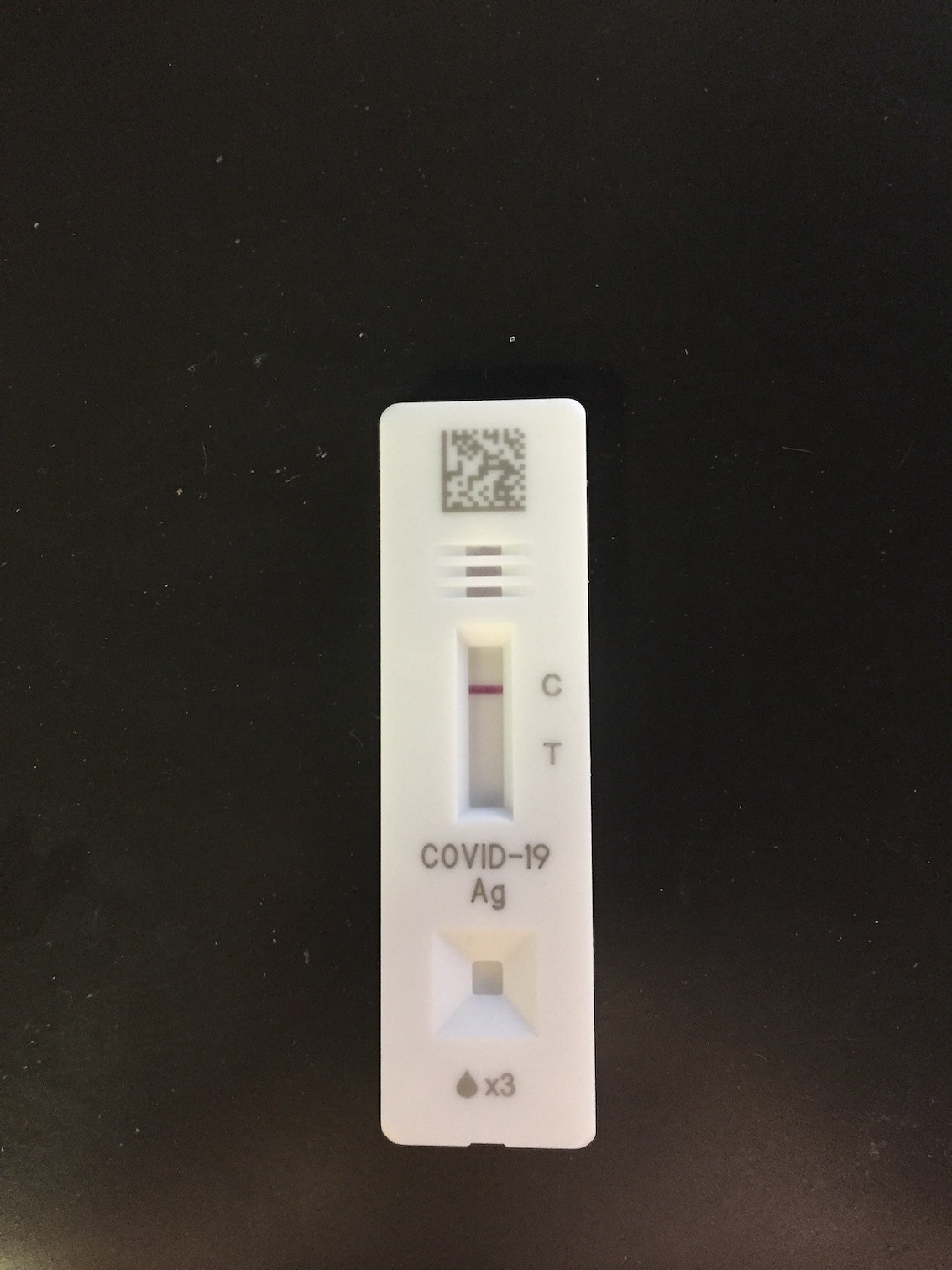The image features a long, thin rectangular COVID-19 rapid test strip made of plastic. The strip displays a barcode at the top, followed by the text "COVID-19 AG" in the middle section. Just beneath this, a transparent section is visible, showing lines and indicators for testing. To the right of the transparent section, the letters "C" and "T" are printed on the plastic, denoting control and test lines respectively. An indentation at the bottom of the strip serves as the area where the sample is applied. Below this indentation, there is an icon resembling a raindrop, accompanied by a small "X" and the number "3," indicating that three drops of the sample are to be placed here. Currently, a single broad red stripe appears next to the letter "C," suggesting a negative test result. The test strip is centrally positioned, slightly lower than center, against a plain, dark rectangular background.